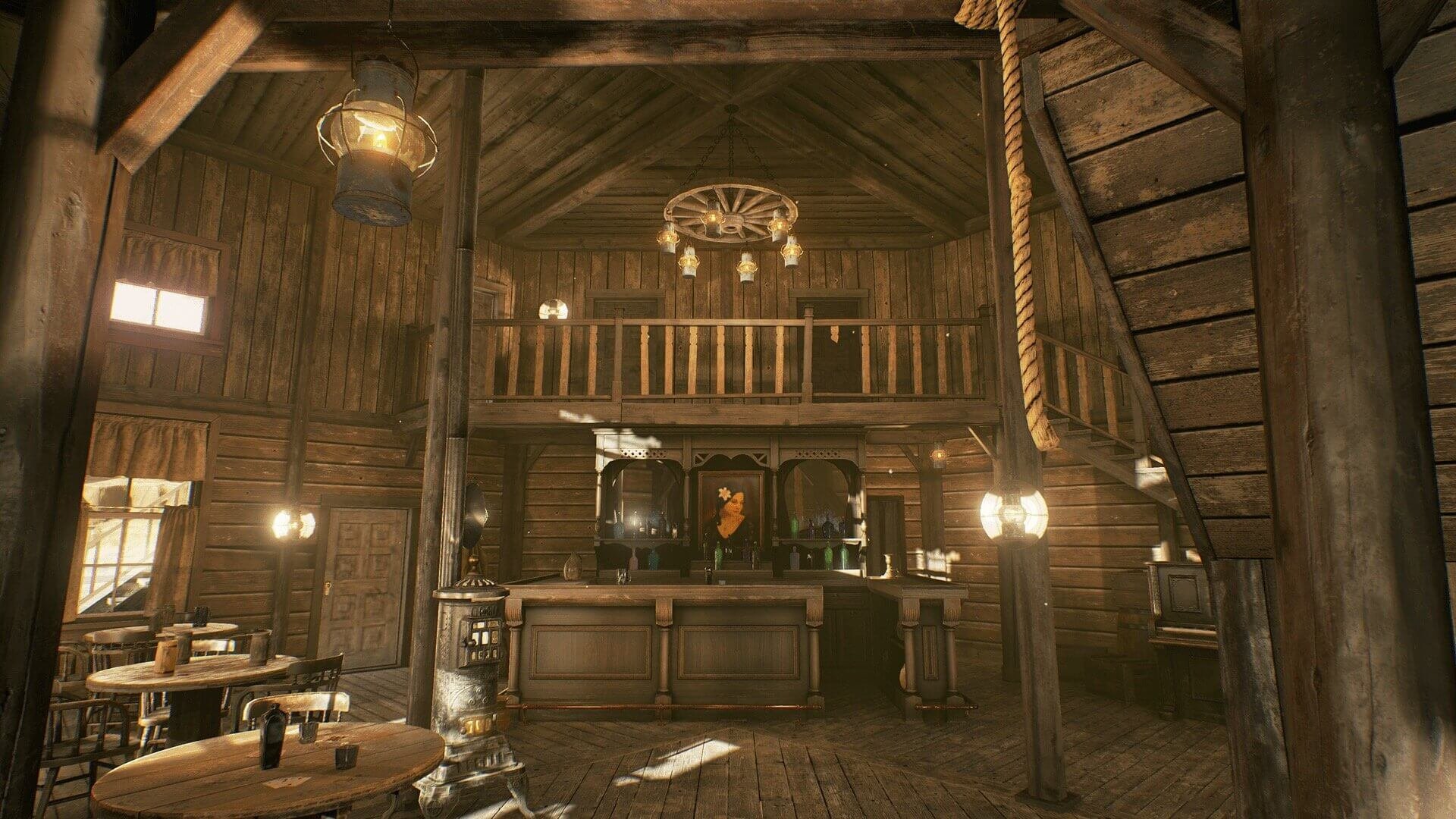The photograph depicts a meticulously detailed computerized rendering of an indoor scene reminiscent of an old Western saloon. The multi-tiered wooden structure features round wooden tables and matching chairs on a wooden floor. Dominating the center is an old-style wooden bar adorned with bottles of various colors including pink, blue, and green. Behind the bar, a portrait of a woman with a white flower in her hair gazes to the right, adding a touch of nostalgic charm. Above, a wide wooden balcony is supported by large wooden posts wrapped with cord, creating a sturdy and rustic atmosphere. A wagon wheel chandelier with smaller period lanterns hangs from the exposed wooden ceiling. Additional lighting is provided by old lanterns suspended from posts and a large rope hanging from the ceiling. The room is framed with small rectangular windows to the left, a wooden door, and an array of iconic Western features such as an antique wood stove, enhancing the tavern-esque ambiance.